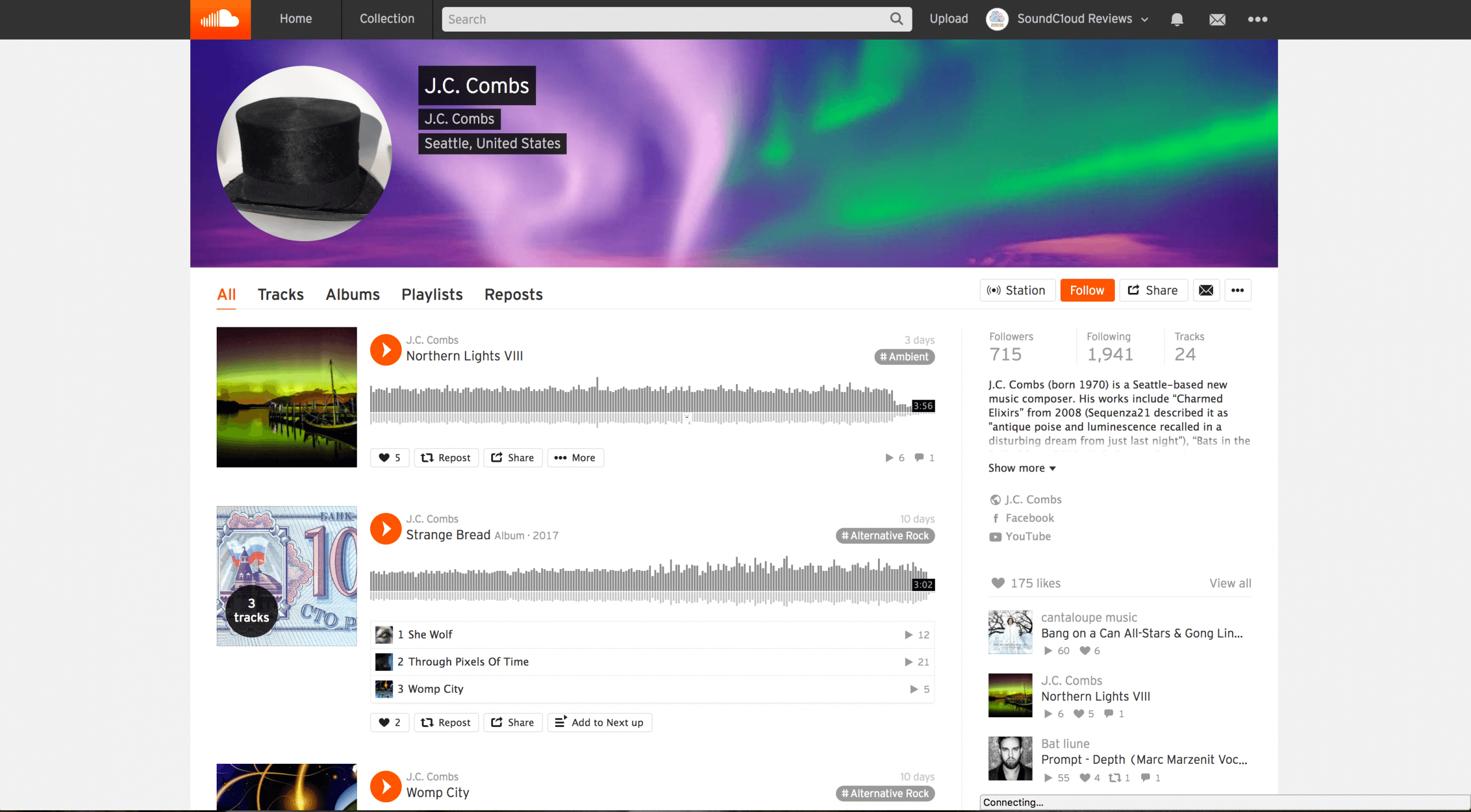Here is the cleaned-up and detailed caption:

---

The image shows a SoundCloud profile page open on a laptop, specifically focusing on the account of JC Combs from Seattle, United States. The profile picture of JC Combs is distinctive, featuring a bowler hat instead of a traditional face image. 

At the top of the profile, major sections such as 'All Tracks,' 'Albums,' 'Playlists,' and 'Reposts' are easily visible. Below these tabs, individual tracks are displayed with a waveform graph shown alongside each track, indicating audio activity as the track plays along its timeline.

The first track listed is titled "Northern Lights," accompanied by a thumbnail depicting the mesmerizing Northern Lights over a river adorned with boats. Adjacent to this, there appears to be some currency representation, showing "10" in large digits, hinting at either a price or a related monetary note.

Further down the profile, the user has a collection titled "Strange Breed." Next to this track, there are performance metrics, including the number of plays, likes, and shares, which can be seen. The profile summary reveals the total number of followers JC Combs has, along with the number of tracks and a follow button for new listeners to join.